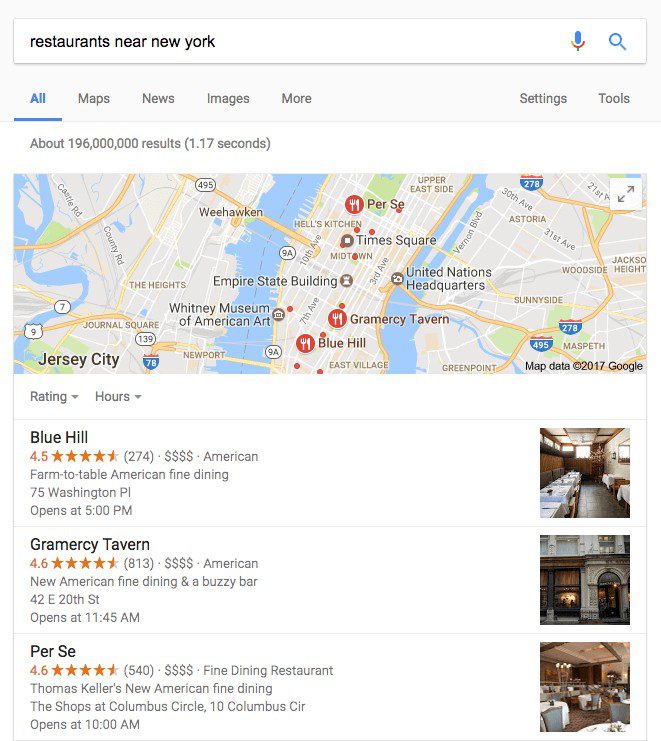The image has a light gray background featuring a search bar at the top with the text "restaurants near New York." The search bar also includes icons for a microphone and a magnifying glass. Below the search bar, there are tabs labeled "All," "Maps," "News," "Images," and "More." On the right side, there's a section for "Settings" and "Tools."

Beneath this interface, a white area displays the search results, indicating about 196 million results were found in 1.17 seconds. The first result shows a Google Maps image of the New York area, highlighting prominent landmarks such as Times Square, the United Nations, the Empire State Building, and the Whitney Museum of American Art.

Directly below the Google Maps image, there is an area that provides ratings and hours for various restaurants. The featured listings include:
1. Blue Hill: Rated 4.5 out of 5 stars based on 274 ratings, categorized under American, farm-to-table fine dining, located at 75 Washington Place, and opens at 5 p.m.
2. Gramercy Tavern: Rated 4.6 out of 5 stars, also noted with four dollar signs indicating a higher price range.